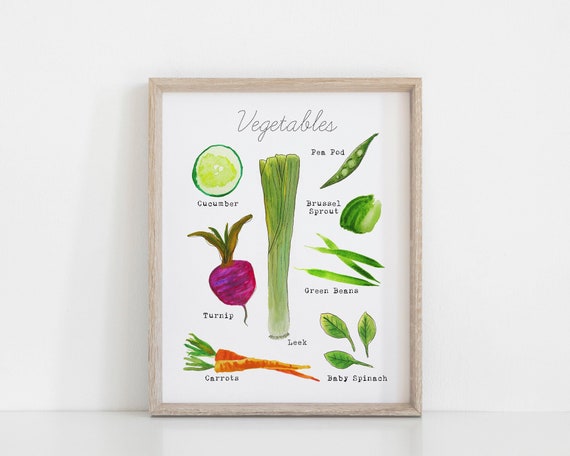This image depicts a vertically rectangular, multi-color artistic print framed in a brown wooden frame without a border, resting on a white countertop against a white wall. The centerpiece of the print is a large green leek located in the center. At the top, in cursive black letters, it reads "Vegetables." The left side from top to bottom features a cucumber, a purple turnip, and a pair of carrots. The right side from top to bottom shows a pea pod, a Brussels sprout, three green beans, and three leaves of baby spinach. Each vegetable is meticulously labeled with its name, all set against a white background. The photograph was taken indoors using artificial light, capturing the vibrant hues of green, orange, light purple, and other earthy tones of the depicted vegetables.